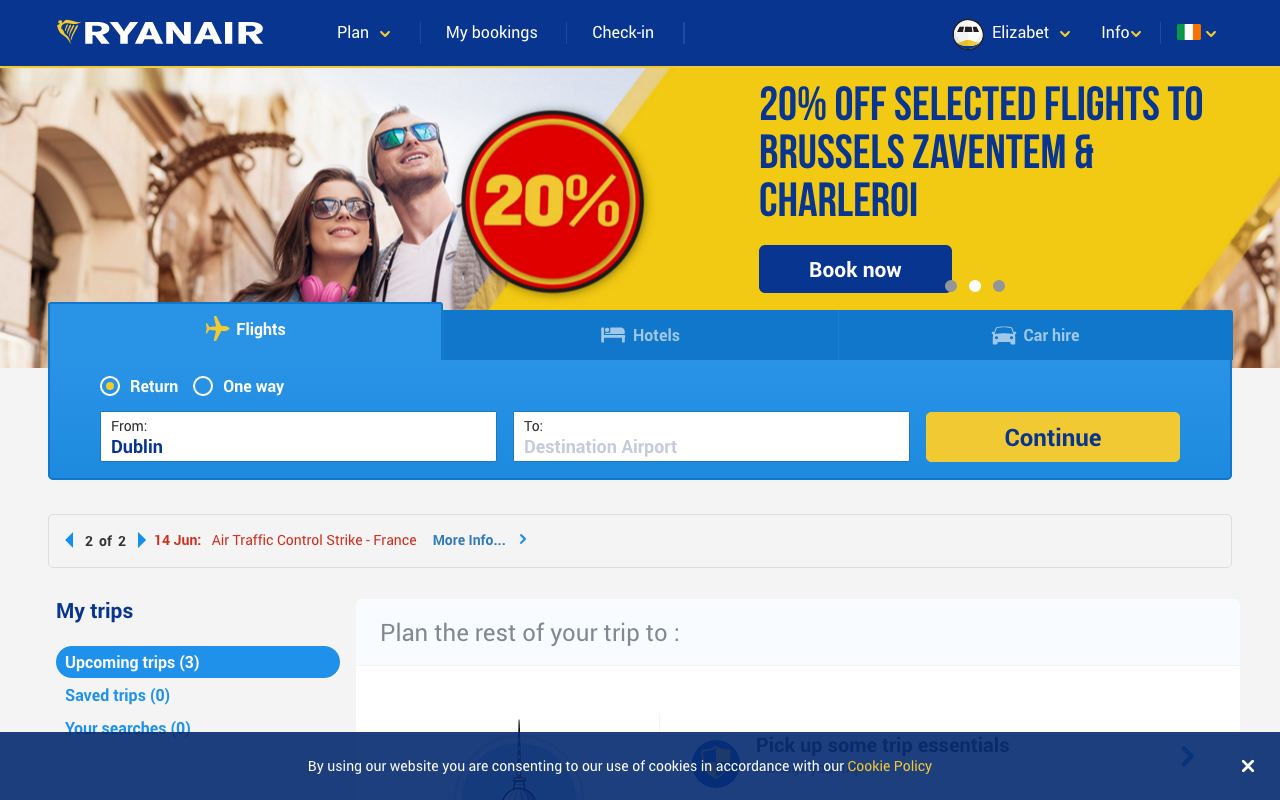The image features a Ryanair web interface with a distinctive blue border at the top. "RYANAIR" is prominently displayed in white capital letters. On the upper right side of the interface, there’s a drop-down menu labeled "Plan." Adjacent to it, tabs labeled "My Booking," "Check-In," "Elizabeth," "Info," and an Irish flag icon are visible, indicating language settings or a regional site.

Beneath this header, the main section of the image showcases a promotional banner. The banner depicts a man and a woman, both wearing sunglasses and standing outside a historical European building, reminiscent of classic architecture. Central to the banner is a red circular sticker proclaiming "20% OFF." 

To the right, against a vibrant yellow background, blue text announces, "20% off selected flights to Brussels, Zaventem, and Charleroi." Below this promotional text is a blue button labeled "Book Now." 

At the bottom of the image, additional navigational options include tabs for "Flight," "Hotel," and "Car Hire." There are also toggle options for "Return" and "One Way" journeys, providing users with easy access to various booking options.